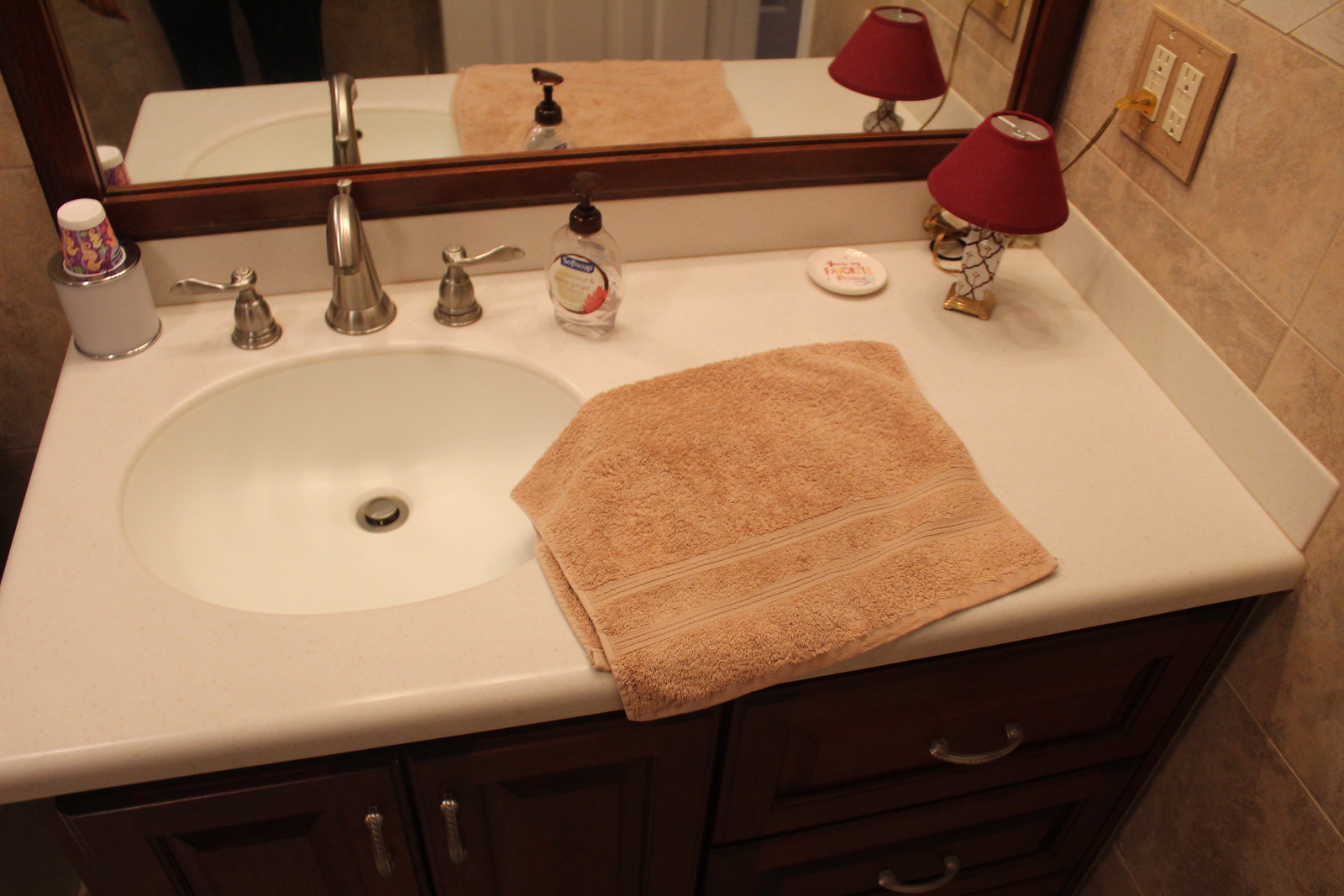The image depicts a well-kept bathroom interior viewed from the perspective of someone standing near the vanity, but slightly off to the side. The setting features a large mirror above a wooden cabinet vanity with drawers and doors beneath a sleek, white marble countertop and integrated sink. Brushed steel knobs adorn the cabinetry, adding a modern touch. To the side of the sink, there's a whimsical paper cup dispenser, likely intended for children, as suggested by the playful cartoons decorating the cups. A bottle of soft hand soap is conveniently placed beside the sink. The ambient lighting lends a warm, pinkish-yellow glow to the space, complementing the predominantly beige, marble-tile wall adorned with subtle earth tones. A small lamp plugged into an outlet on the opposing wall adds a cozy and functional element to the overall serene bathroom setting.